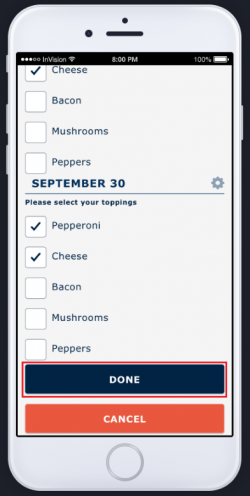In the image, a modern, large white cell phone is prominently displayed against a solid black background. The phone screen shows a detailed list, resembling a digital interface, possibly for ordering pizza. At the top of the screen, there is a dark status bar showing various icons: cell signal strength, an "InVision" logo, Wi-Fi signal, the time (8 PM), and a 100% battery indicator.

Below the status bar, the screen transitions to a predominantly white background with a clear checklist layout. The checklist allows users to select pizza toppings, with small checkboxes aligned to the left of each topping: 

1. Cheese (checked)
2. Bacon (unchecked)
3. Mushrooms (unchecked)
4. Peppers (unchecked)

Further down, the interface displays the date "September 30" and a settings icon to its right. The instruction "Please select your toppings" appears above the checklist, guiding the user on what actions to take. The list includes:

- Pepperoni (checked)
- Cheese (checked)
- Bacon (unchecked)
- Mushrooms (unchecked)
- Peppers (unchecked)

At the bottom of the screen, there are two buttons for confirmation: a blue "Done" button outlined in red, with white text, and a red "Cancel" button with white text. These elements suggest a user interface, potentially part of an educational tool or interactive tutorial for placing an order online, possibly for a restaurant setting. The meticulous design and instructional text imply this might be a demo for a website or an app, guiding the user through the process of customizing a pizza order.